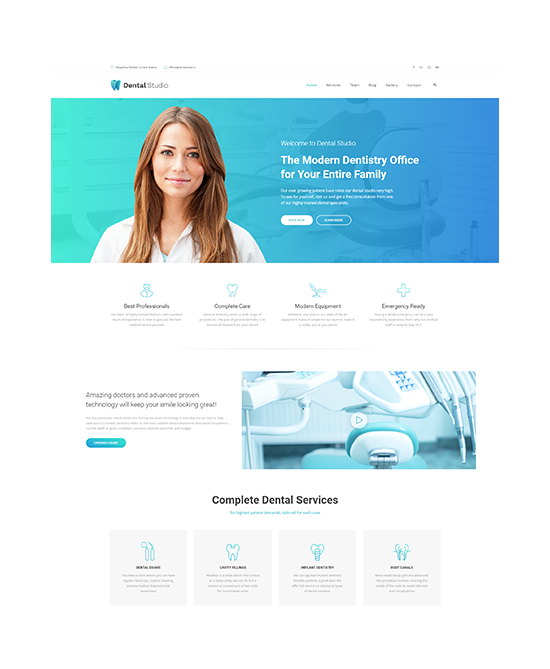The image depicts a dental studio's website interface. In the upper left corner, there is a label that reads "Dental Studio." The top right corner features a navigation menu, but due to poor resolution, the menu text is unreadable. Below the header is a horizontally elongated rectangle showcasing a portrait of a woman. The photograph captures her from just below the shoulders upward. She has long, dark brown hair and a tan-pink complexion. The woman is smiling directly at the viewer.

To the right of her, the text reads, "Welcome to Dentist Studio, the modern dentistry office for your entire family." More text appears underneath, but it is too small to discern. There are also two buttons below this text— one white and one blue— both of which are unreadable.

The background behind the woman's image transitions from green on the left to blue on the right. Below this main image is a photograph that displays the colors green and blue, featuring a dentist's chair and a worker's chair.

Further down, there are phrases indicating professional services, such as "complete care," "modern equipment," and "emergency ready." Another section mentions "amazing doctors" and "advanced technology" that are dedicated to maintaining a great smile.

At the bottom part of the image, there is a segment titled "Complete Dental Services." This section contains four boxes, each with a blue icon, a black header, and a short paragraph of text, all of which are unreadable due to the poor resolution.